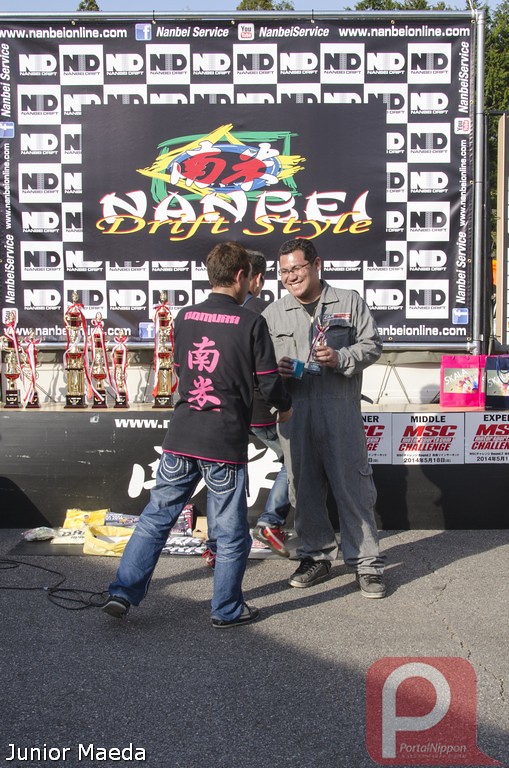The photograph captures a vibrant and festive celebration ceremony taking place outdoors on a makeshift stage set up in a parking lot. Central to the image are two men standing in front of the stage, engaged in a firm handshake. The man on the left is dressed in blue jeans paired with a traditional Japanese jacket adorned with distinctive character symbols down the back. On the right, the other man is clad in gray coveralls, reminiscent of a mechanical jumpsuit, and he proudly holds a trophy, indicative of an award he has won.

The stage behind them is decorated with a variety of trophies, each embellished with white and red ribbons, alongside numerous gift bags and promotional items that underline the event's celebratory nature. A striking black backdrop stretches across the stage, prominently featuring a logo composed of an N and a D, flanked by white writing that reads "N-A-N-B-E-I online dot com" and "NANBAI service," which repeats around the border. A central black rectangle on the backdrop displays vibrant colors—yellow, white, red, blue, and green—and the words "NANBAI" and "drift style" in a Japanese-style font.

Further adding to the backdrop's detail, "Junior Media" is inscribed on the left side, while a red square with a white P is visible on the right. The scene exudes a sense of accomplishment and festivity, capturing a moment of recognition and celebration amidst the detailed cultural and promotional display.